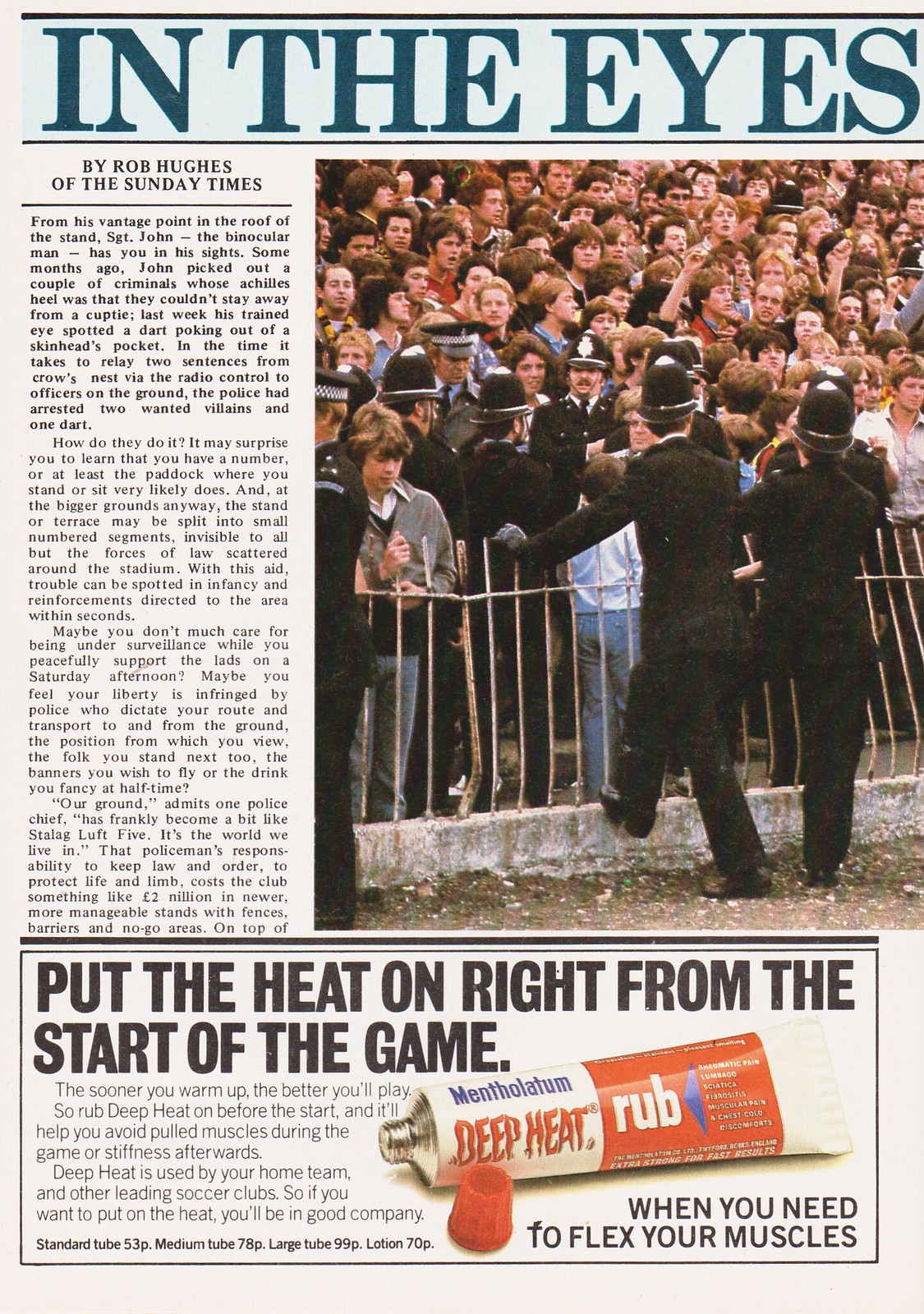This image, likely from a magazine or newspaper, features an article titled "In the Eyes" by Rob Hughes of the Sunday Times, set in prominent blue letters at the top against a light blue background, bordered by black bars. The article's main narrative, in bold text, recounts the vigilance of Sergeant John, dubbed "the binocular man," who monitors a crowd from the roof of a stand. Previously, his keen observations led to the arrest of criminals fixated on a "cup tea," and recently, he noticed a dart in a "skinhead's pocket," resulting in swift police action leading to arrests.

The article explains the surveillance tactics at large stadiums, including numbered seating sections only identifiable to law enforcement to curb trouble early and efficiently. This protective measure, despite seeming like an infringement on personal freedom, is deemed necessary by law enforcement, costing clubs around two million pounds annually.

Adjacent to the text is a photograph showing British police officers standing in front of a fence, containing a sizable crowd gathered behind them. At the page's bottom is an advertisement for Methyl Latium Deep Heat Rub, emphasizing the phrase "Put the heat on right from the start of the game," with the image of the product tube. The ad promotes the rub as essential for muscle relaxation, preventing strains, and easing stiffness, endorsed by leading soccer clubs.